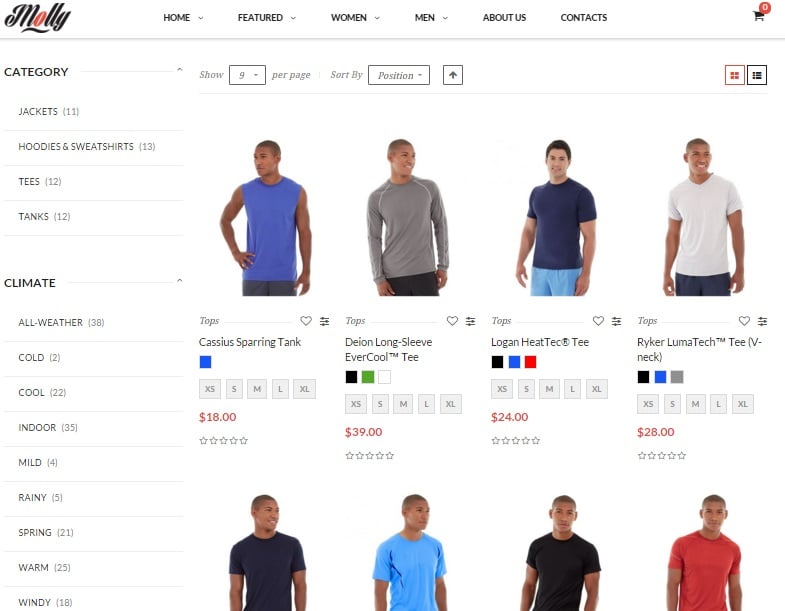A screenshot from an e-commerce website specializing in t-shirts is displayed with a predominantly white background. In the upper right corner, a black shopping cart icon is shown with the number "0" next to it, indicating no items in the cart. The upper left corner features the brand name "MOLLY," where the letter "O" is highlighted in red and the rest of the letters (M, L, L, Y) are in black. The primary navigation menu includes options labeled: HOME, FEATURED, WOMEN, MEN (each with drop-down selections), ABOUT US, and CONTACTS.

On the left side of the screen, a detailed category list appears, labeled "CATEGORY," followed by subcategories: JACKETS (11), HOODIES AND SWEATSHIRTS (13), TEES (12), and TANKS (12). Below this, a section titled "CLIMATE" lists various weather-appropriate clothing options: ALL WEATHER (38), COLD (2), COOL (22), INDOOR (35), MILD (4), RAINY (5), SPRING (21), WARM (25), and WINDY (18).

To the right of the categories, there is a selection box that says "SHOW 9 PER PAGE" with a drop-down menu and sorting options labeled "SORT BY POSITION" with an accompanying up arrow. There are also GRID and COLUMN view selection buttons, with the GRID view currently active.

The main content area features images of young men modeling various t-shirts in colors like blue, grey, navy, white, sky blue, black, and red. Each shirt is listed with its name and price: Cassius Sparring Tank ($18), Dion Long Sleeve Evercool Tee ($39), Logan Heat Tech Tee ($24), and Riker Luma Tech Tee V-Neck ($28).